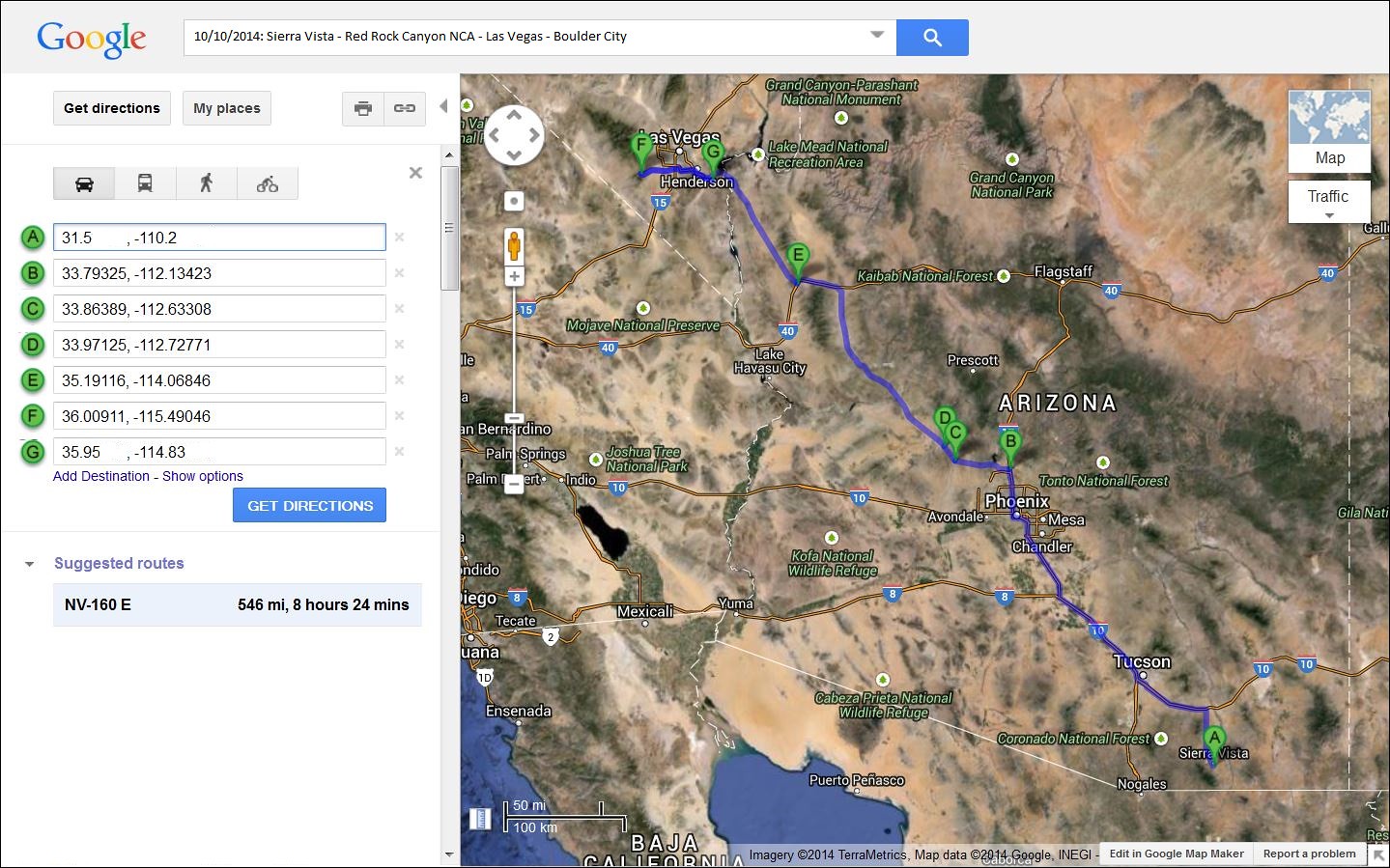This image is a screenshot from Google Maps, illustrating a planned road trip. The itinerary begins in Sierra Vista, continues to Red Rock Canyon, and proceeds to Las Vegas, Nevada. The route then heads to Boulder City before traveling down to Tucson, Arizona, and ultimately circles back to Sierra Vista. The map highlights the entirety of the selected driving route, which is estimated to take 8 hours and 24 minutes. Various waypoints are marked to show significant stops along the journey. The user seems to be utilizing the route planning feature of Google Maps to organize this extensive trip, showcasing a detailed itinerary and travel duration.